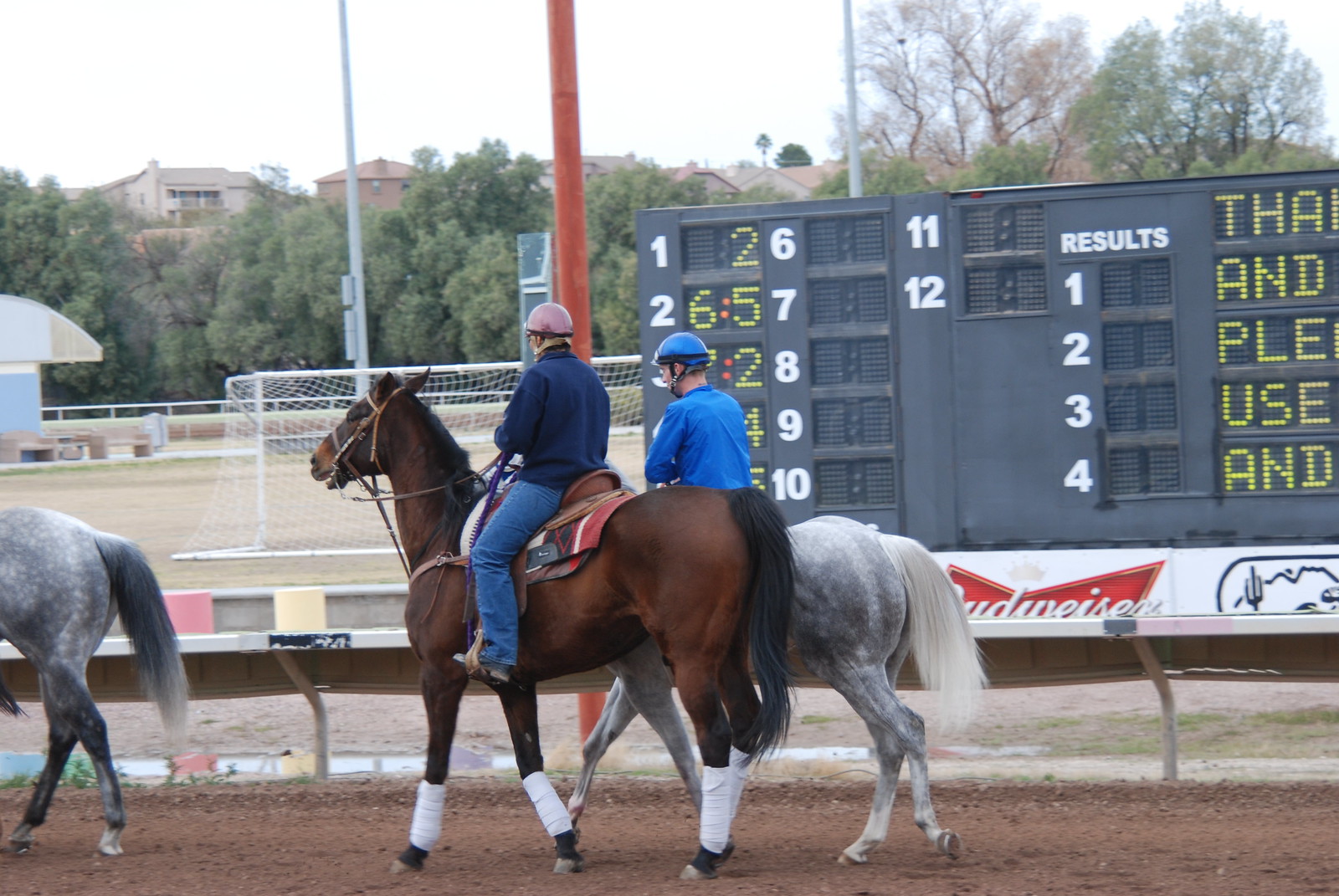In this landscape-oriented image, two jockeys are riding horses side by side on a brown dirt racetrack, heading to the left in a side profile view. Leading the pair is an older man on a brown horse with white leg wraps, dressed in a helmet, jeans, and a dark blue sweatshirt. Following closely is another jockey wearing a blue helmet and a light blue shirt, mounted on a dapple gray horse. Behind them, an electronic scoreboard displays horses' names and betting odds. The track is bordered by a fence, and in the background, there is a soccer field with a visible net, several homes, trees, and utility poles. The horses appear to be walking or trotting, either preparing for or cooling down from a race.